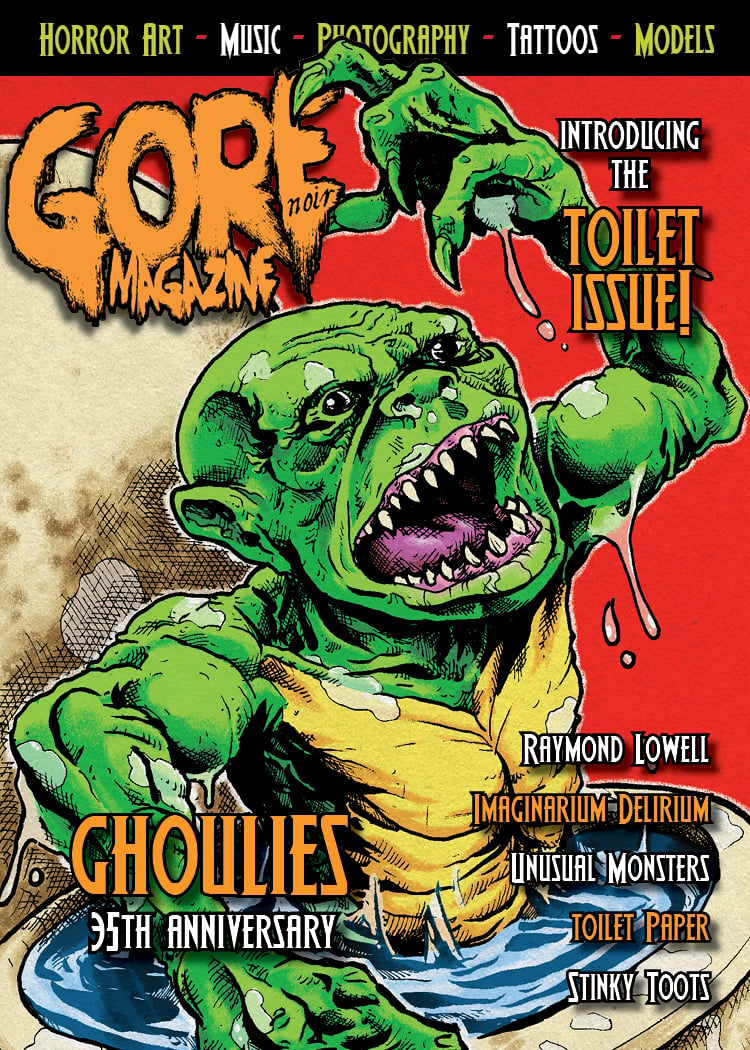The magazine cover promotes the 35th anniversary of "Ghoulies" in Gore Noir Magazine. At the top, a bold black stripe features the words "HORROR ART – MUSIC – PHOTOGRAPHY – TATTOOS – MODELS" in alternating yellow and white text. "GORE NOIR MAGAZINE" is written in gory orange letters on the top left, and to the right, "Introducing the Toilet Issue" is prominently displayed.

Dominating the center is a striking image of a green creature that resembles an ogre or swamp monster. It has a bald head with large black eyes, sharp white teeth set in pink gums, and a purple mouth, wide open as if growling. The monster emerges from a pool of water or goo, which is dripping off its muscular arms and sharp-clawed fingers. It appears to be wearing a yellow vest-like shell. 

The bottom left corner of the cover celebrates "Ghoulies' 35th Anniversary," while the bottom right lists additional features: "Raymond Lowell, Imaginarium Delirium, Unusual Monsters, Toilet Paper, and Stinky Toots." The overall design has a graphic novel or comic book style, enhancing its eerie and fantastical theme.